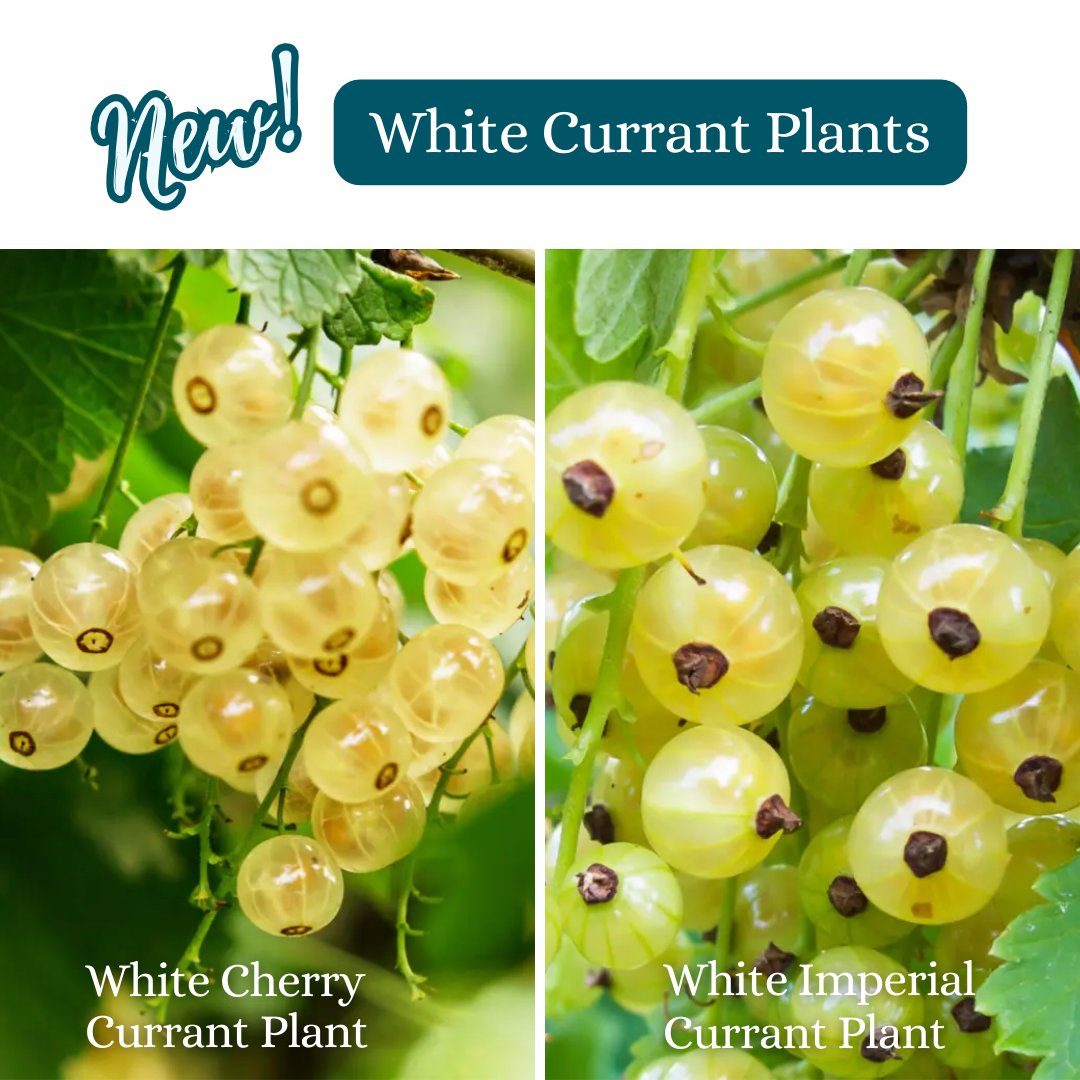The image showcases two photographs side-by-side against a white background, labeled "new" in script letters, with a dark teal stripe above bearing the title "White Currant Plants" in white, serif text. Each photograph features a close-up of white currants still on the bush, set against a green background, capturing clusters of small, spherical berries with a translucent and glistening appearance. The left photograph, labeled as "White Cherry Currant Plant," depicts currants that are very light green to a light yellowish color, with round brown bases at the tips. The right photograph, labeled "White Imperial Currant Plant," shows slightly larger currants that have light green lines with more pronounced brown stems. Both varieties are similar in their grape-like, spherical shape and translucent, greenish hue, highlighting subtle differences in coloration and stem prominence.